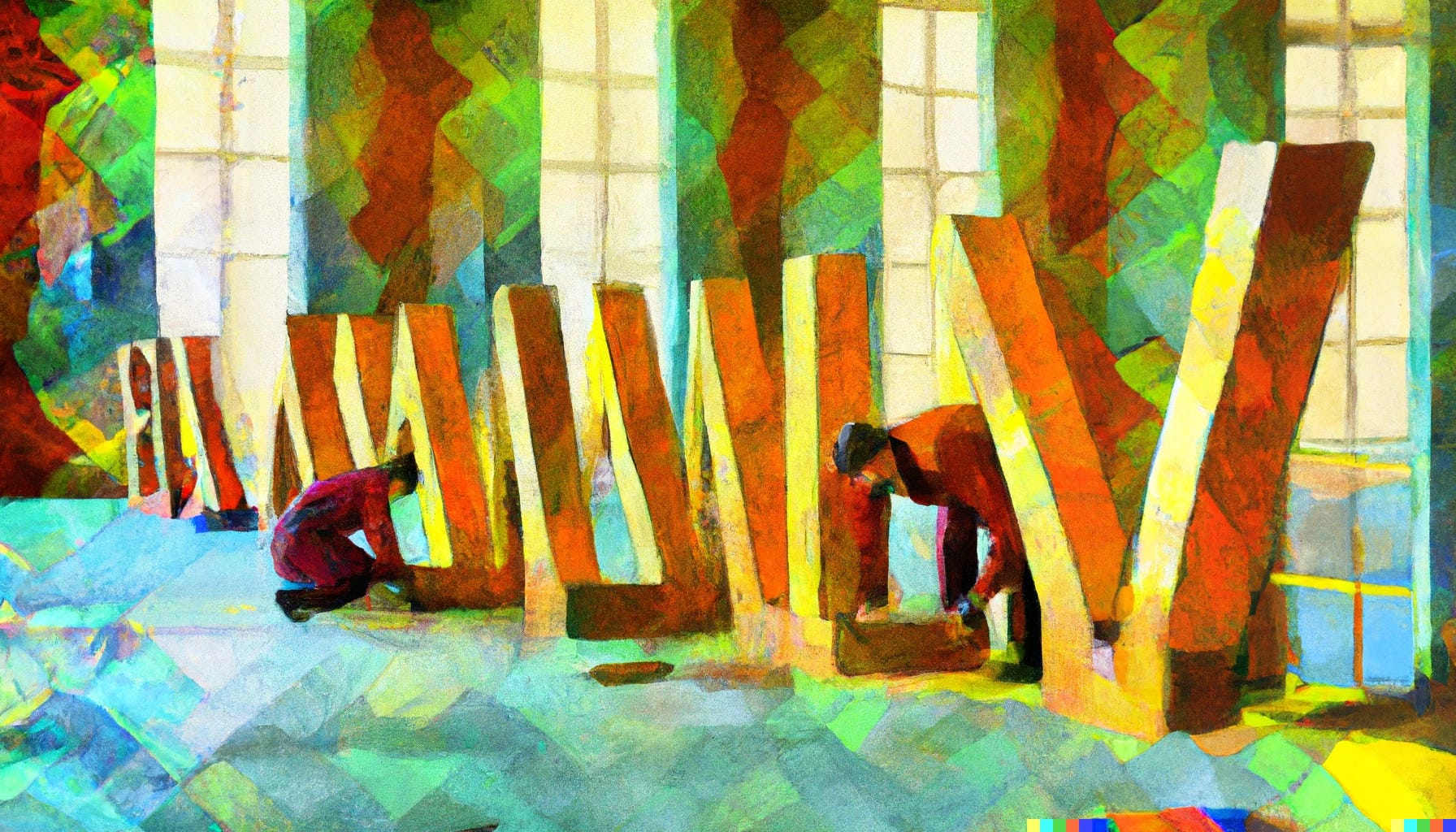This horizontally aligned, borderless painting depicts an indoor scene characterized by its vivid colors and geometric designs. The floor is adorned with colorful geometric shapes, including squares and diamonds, creating a vibrant base for the artwork. Prominently featured are large block letters, with visible characters such as V, L, M, and A, though the exact arrangement is ambiguous. Two men, appearing to be workers, are engaged with these letters—one on the left and one on the right—seemingly positioning them. 

In the background, vertical strips of windows alternate with bright, multicolored walls decorated with geometric patterns in green, red, blue, yellow, and triangular designs. These windows repeat in different rows, adding depth to the scene. The entire composition is bathed in tones of green and red, highlighting the lively and abstract nature of the painting. Overall, it presents a dynamic and busy scene within a colorfully adorned room.